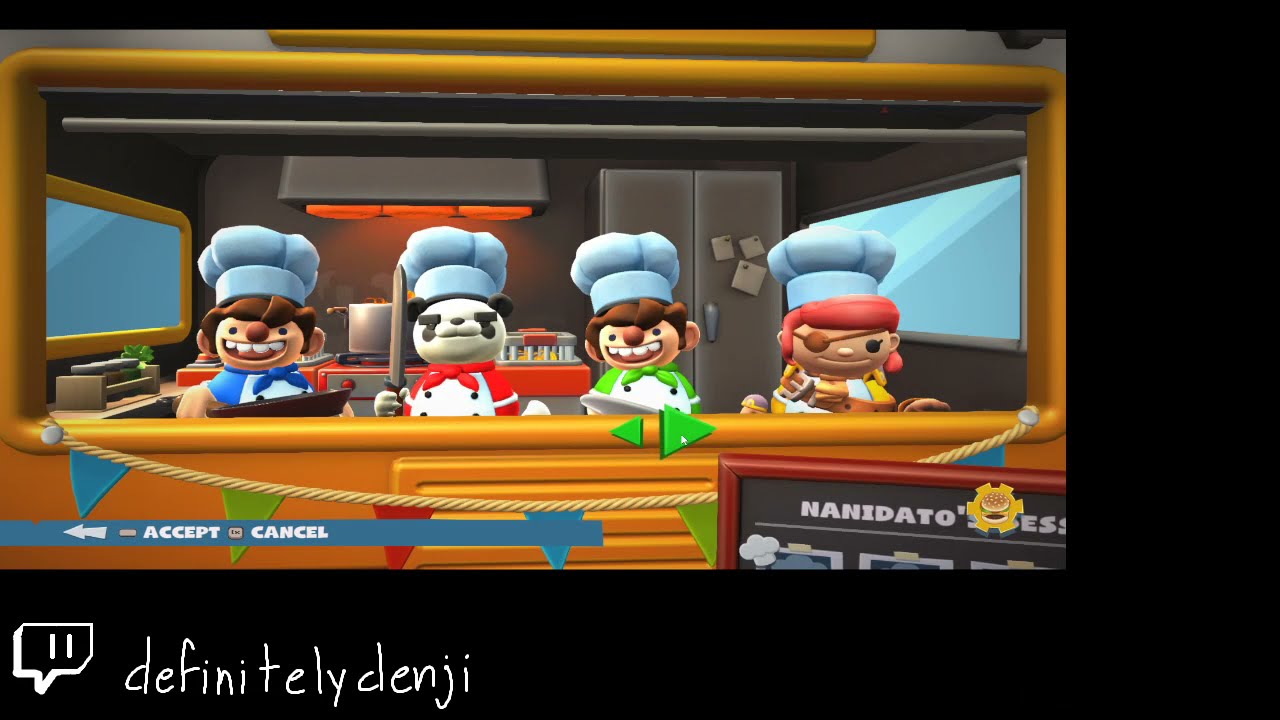In this colorful and vibrant screenshot from a video game reminiscent of "Overcooked," four cartoon characters are captured in a bustling restaurant kitchen scene, situated in the upper left-hand corner of the image. Each character is adorned with a chef's hat, emphasizing their culinary roles. From left to right, we see a cherubic pair of identical twins flashing goofy smiles, donning colorful aprons and bow ties. Next is a character with distinctive red hair and an eye patch, possibly named Nana Dado, as indicated on a chalkboard beneath them. 

The fourth character is an adorable panda bear, uniquely brandishing a sword. The panda is dressed in a red coat and bow tie, and stands out with its whimsical juxtaposition of a chef’s attire and adventurous weapon. The kitchen background includes a visible commercial stove with a pot, a refrigerator, and a large window on the right-hand side, adding to the lively restaurant atmosphere.

Below this lively scene, in the bottom left-hand corner of the image, the text "definitely denji" appears, resembling handwritten script, hinting that this is a screenshot from a Twitch stream. The distinctive thinness of the font and variances in repeated letters like "D," "E," and "I" suggest a personalized touch, enhancing the overall charm of this delightful kitchen setup. The image is framed with a black border along the right edge and bottom edge, adding a finishing touch to this captivating snapshot.